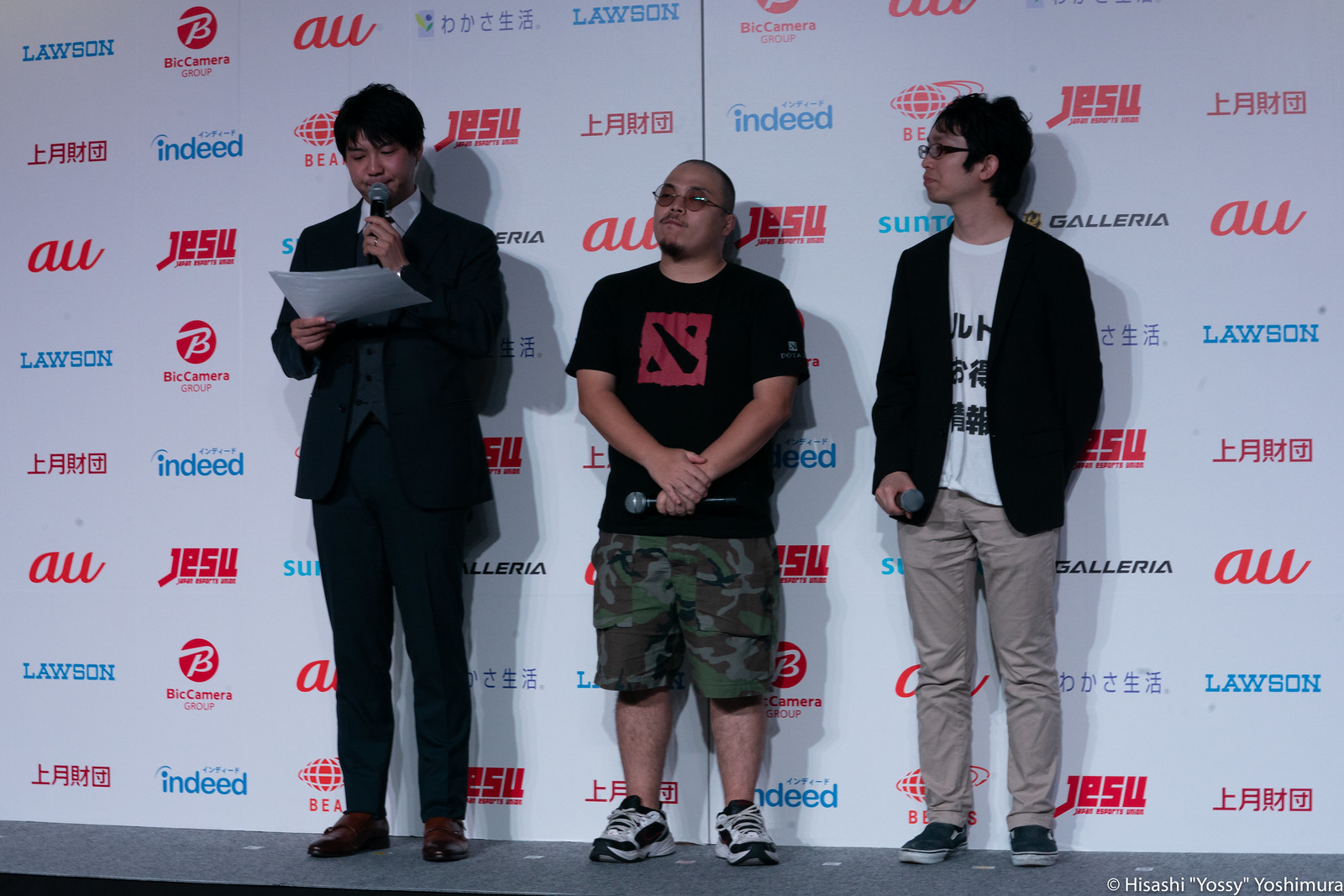This image depicts three men standing on a stage in front of a backdrop adorned with various sponsor logos, including Lawson, Indeed, Jesu, Bic Camera Group, AU, and Galleria, along with others in an Asian script. The backdrop primarily features blue, black, and red text on a white background. 

The man on the left is dressed in a full three-piece suit with brown shoes and has messy hair. He holds some papers in one hand and a microphone in the other. The man in the middle, who has a shorter stature, is wearing a black Dota 2 t-shirt featuring a red graphic, camouflage shorts, sunglasses, and sneakers. He stands with his hands clasped in front of him, holding a microphone in one hand. The man on the right is sporting a casual look with a black open cardigan over a white t-shirt that has Asian lettering on it, khaki pants, sneakers, and dark-rimmed glasses. All three individuals appear to be Asian, and they are likely part of some kind of presentation or event, given their stage setting and professional to semi-casual attire.